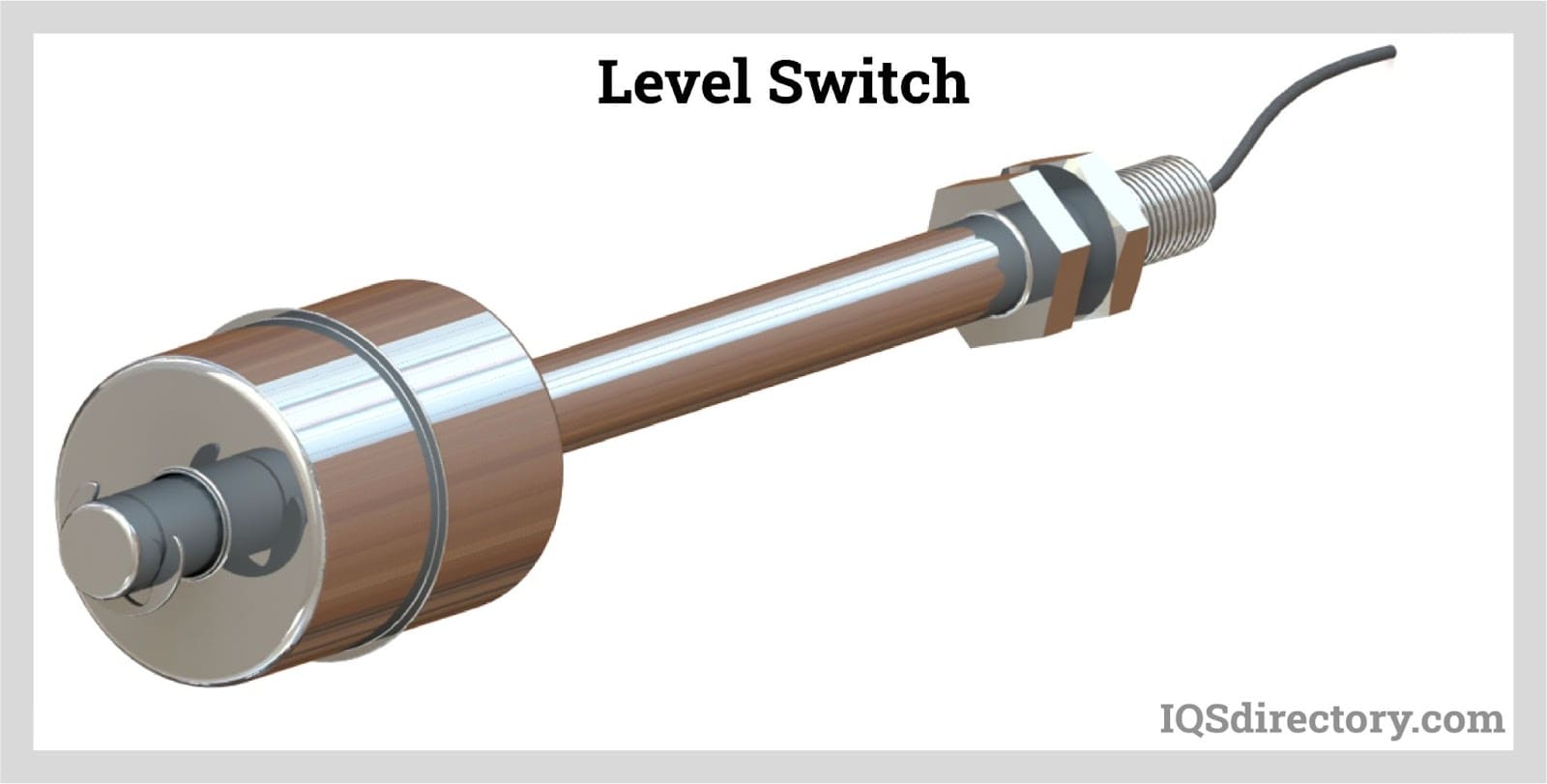The image showcases an illustrated tool known as a level switch, prominently labeled "Level Switch" at the top in black letters. The tool itself is constructed from steel and features a screw base from which a metal wire extends. This wire connects to a rod topped with thick washers, resembling a small barbell or dumbbell. The assembly includes wing nuts on the screw portion, adding to its functional design. The tool is depicted against a white background, bordered by a rectangular gray edge. At the bottom right of the image, the source is indicated as "IQSDirectory.com," suggesting the illustration is featured on their website.